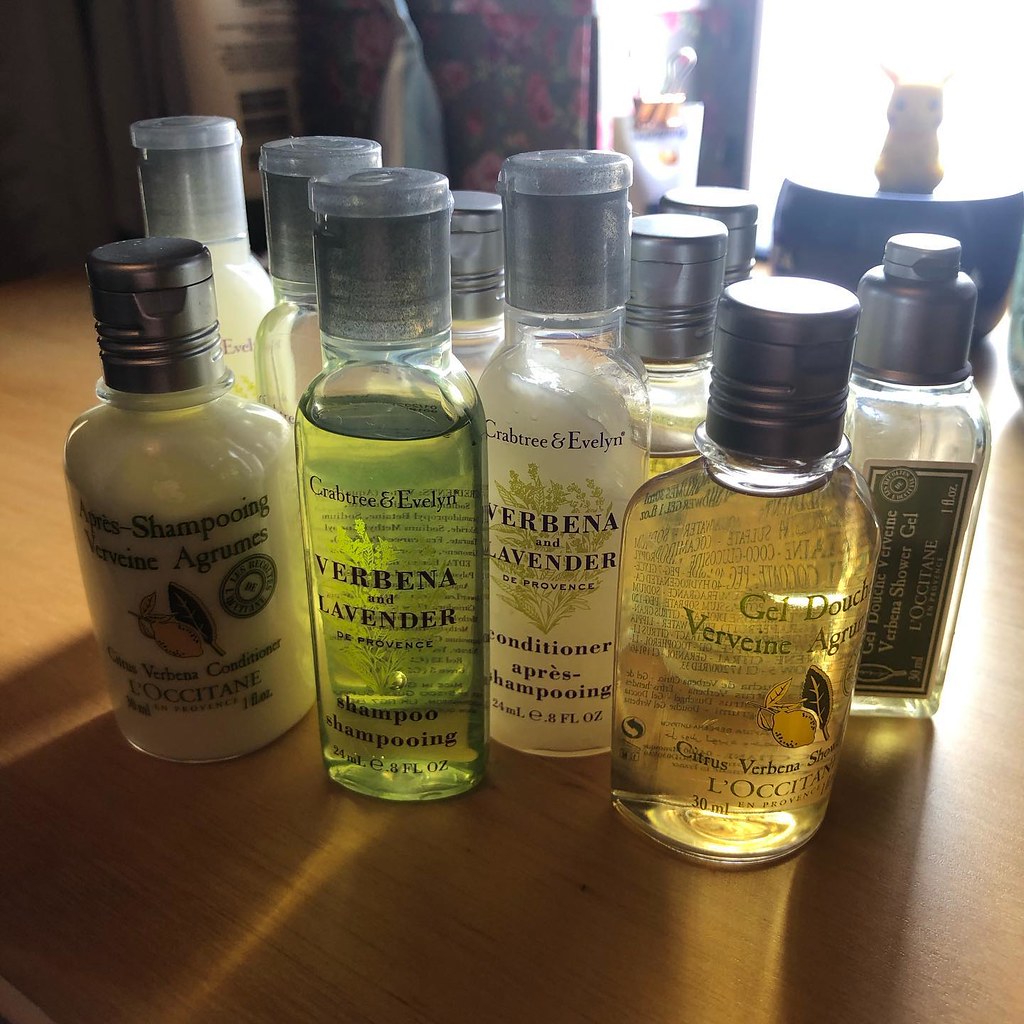In this image, a neatly arranged collection of personal care products rests atop a brown countertop. The products, primarily from the brands Crabtree & Evelyn and L'Occitane, include bottles of various shampoos, conditioners, body washes, and shower gels. These bottles feature grey lids and labels with predominantly black text. The containers appear to be made of either plastic or glass and are transparent, revealing the diverse colors of the contents inside: a green liquid, a creamy white substance, and a yellow, gel-like solution. This scene appears to be set in a bathroom, and in the background, near a window, there is a yellow Pikachu toy, adding a whimsical touch to the pristine arrangement.